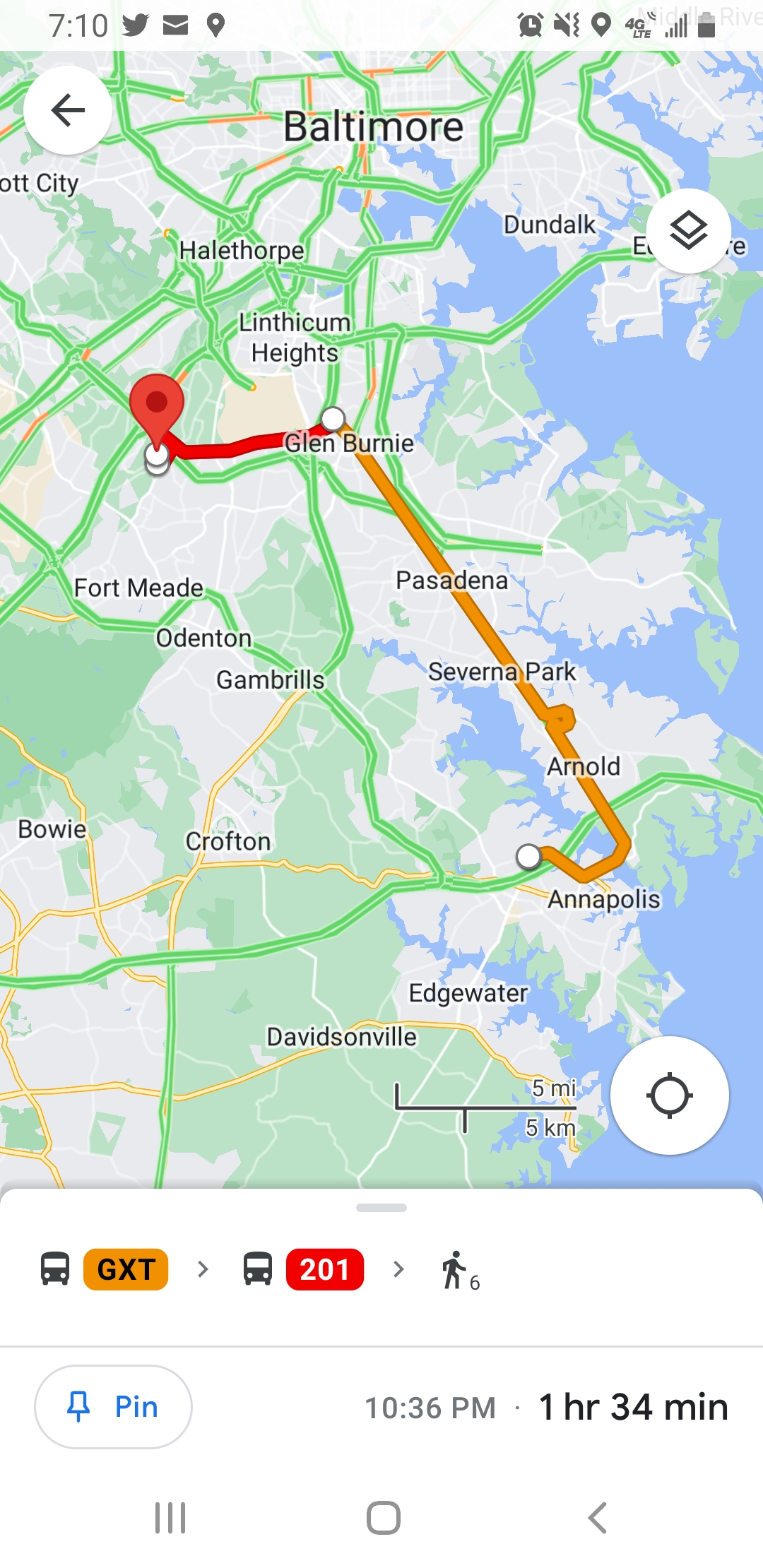This screenshot from a smartphone depicts a detailed route on Google Maps for a journey across Maryland. The map highlights major areas including Baltimore at the top, and suburbs like Dunlap, Heathrow, and Acadium Heights. Icons from the phone interface, such as the time (7:10 AM) and connection details (4G LTE, full service bars, partially depleted battery), are visible at the top. The journey starts in Annapolis, marked in yellow, and proceeds northward towards Baltimore with final stops in its suburbs, using a combination of two bus routes (GXT in yellow and 201 in red) and a walking segment, as indicated by the corresponding symbols. The total travel time is shown to be one hour and 34 minutes. The route is visually represented with colored lines: orange indicating the current travel path and red for the final destination marker.